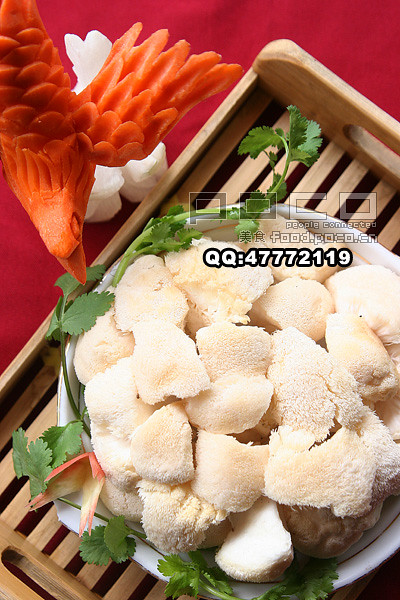The image features a detailed and intricately arranged setting. At the center of the scene, there's a circular dish placed inside a wooden tray. The dish appears to contain a food item that resembles a light-colored or white mushroom or fungus, possibly cauliflower. This central item is surrounded by various garnishes, including greens that look like coriander on a vine and a fruit skin carved intricately. The right side of the tray has an elaborate bird sculpture, which seems to be made from either butter, soap, or carved from a carrot, highlighting its fine details, especially in its wings. The background of the image displays a rich red fabric, potentially a tablecloth, adding a vibrant contrast to the overall earthy tones of the tray and dish. The setting suggests it could be a kitchen or a restaurant. Additionally, the top of the image contains a watermark that reads "Poco, people connected" along with "food.poco.cn" and "qq.47772119."